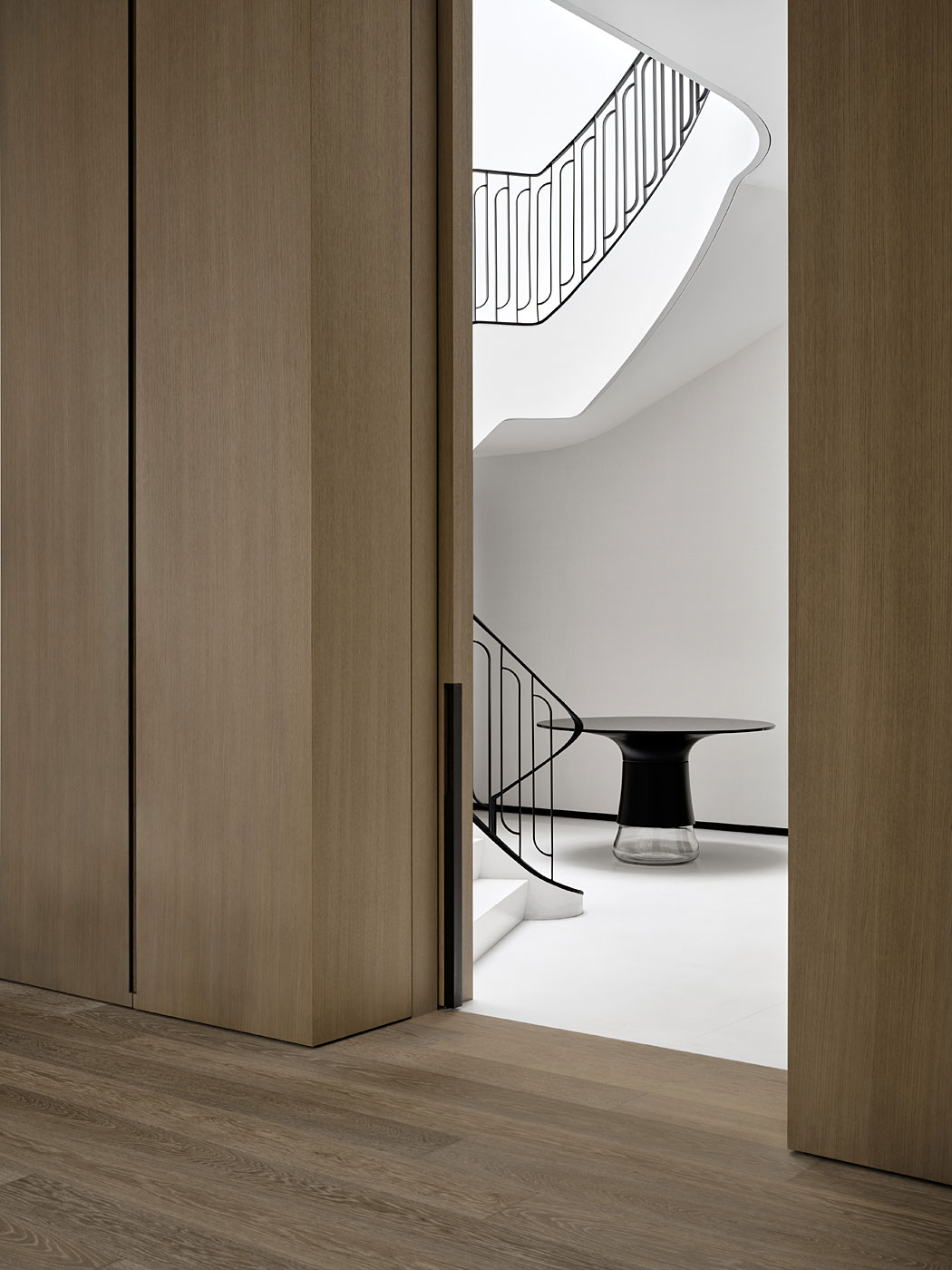This photograph captures the interior of a minimalist building with a stark contrast between two adjoining rooms. The foreground features a room dominated by medium-toned wooden elements, including smooth, thick wooden walls and a hardwood floor. A tall, narrow vertical doorway leads from this wooden room into a pristine, entirely white corridor. Within this corridor, a modern spiral staircase ascends to the right, characterized by thin, abstract-looking black metal railings. At the base of the stairwell sits a distinctive round black table with a clear, likely glass base, adding to the sleek, contemporary feel of the space. Overall, this image exudes a cold, minimalist ambiance, blending the warmth of wood with the starkness of white and black elements.